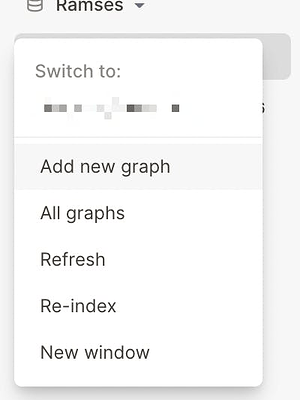A detailed screenshot depicting a dropdown menu within a phone-formatted interface. The menu, titled "Ramses," includes several options, hinting at its likely use in a graphing application. Options listed in the menu are "switch to," followed by an array of various grayscale squares lined up horizontally, suggesting a potential color selection feature. Subsequent options include "add new graph," "all graphs," "refresh," "re-index," and "new window." Notably, the grayscale squares do not follow a linear gradient pattern, indicating they might originally be in color but have been converted to grayscale in this screenshot.

In the background, partially hidden by the dropdown menu, is a rounded gray box, suggesting that a selection action might be taking place. The dropdown menu itself features rounded corners and a drop shadow, enhancing its three-dimensional appearance on the screen.

The header "Ramses" possibly denotes the name of the graph or a related function, accompanied by a partially visible rounded cylinder icon and the top of the name "Ramses" being slightly cut off, with the letter 'R' incomplete. This visual cue implies that either the screenshot cut off part of the header or the interface is adjustable. Overall, the screenshot gives a glimpse into the interface and functionality of an application, likely designed for graphing or data visualization tasks.